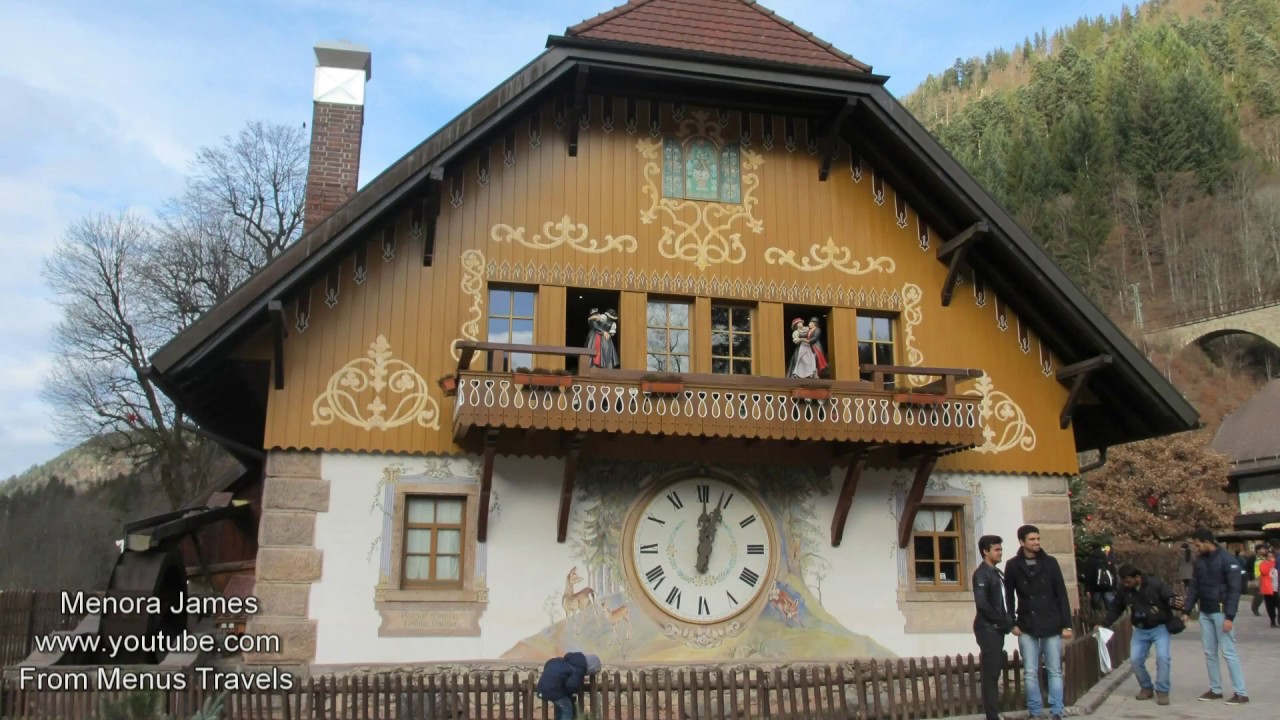The photograph, a vibrant landscape-oriented image, captures a large, house-sized German-style cuckoo clock that resembles a two-story single-family home. The entire front facade of the house is dedicated to the clock and its mechanism, making it a unique tourist attraction located in the Black Forest, Germany. The bottom half of the house is painted white with faux stone bricks at the corners. At the center of the white facade is a large clock face with gray hour, minute, and second hands, and black Roman numerals. Surrounding the clock is a painted woodland scene featuring deer, adding a rustic charm.

Flanking the clock, there are windows with brown wood frames and a prominent balcony above, adorned with animatronic figures that appear to be dancing. A small green door is situated where the cuckoo bird would emerge. The top half of the house features a brown tile roof, accented by a Dutch lap roof and a brownish brick chimney on the left. There's also decorative millwork on a walk-out balcony at the center.

The image shows a bright blue sky with fluffy clouds overhead, surrounded by trees and mountains covered with aspens. The scene includes several tourists and a fence marking the boundaries of the tourist spot. Notably, the bottom left corner of the image displays white text reading "Menorah James www.youtube.com from Menus Travels." The hotel in the photograph is identified as Hotel Hofgut Sternen, blending traditional German architecture with a charming, clockwork attraction.